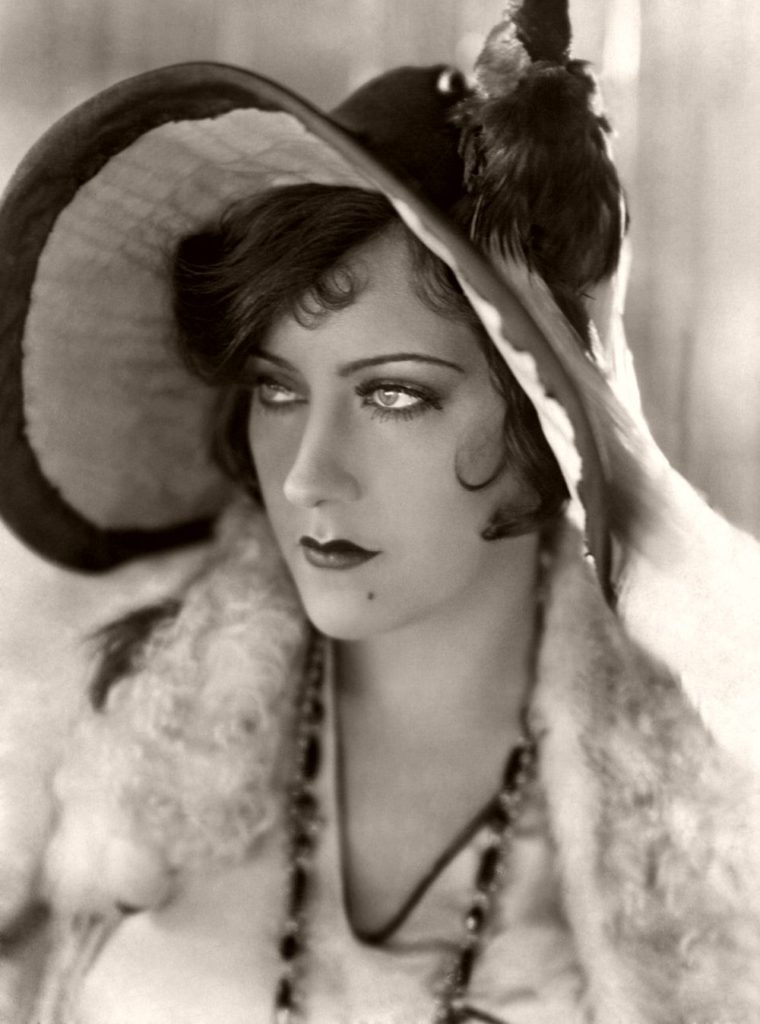In the black and white photograph, a young woman exudes an air of timeless elegance. She is adorned in a large, striking hat with a wide brim that casts a shadow over her face, complete with a black plume of feathers on the crown. Her dark hair, styled in a short, almost page-boy cut with graceful curls framing her face, is complemented by pencil-thin eyebrows and smoky eye shadow. Her pale skin contrasts against dark, likely red lipstick, highlighting her beauty mark situated on her chin beneath her lips. She gazes intently into the distance, exuding an aura of contemplation. She is dressed in a fur coat over a light-colored, gauzy blouse, and a black beaded necklace—possibly accented with gems or jewels—adorns her neck. The photograph's background is a blurry monochrome, possibly depicting a curtain or a wall, ensuring that the viewer's focus remains on her striking visage and vintage attire.